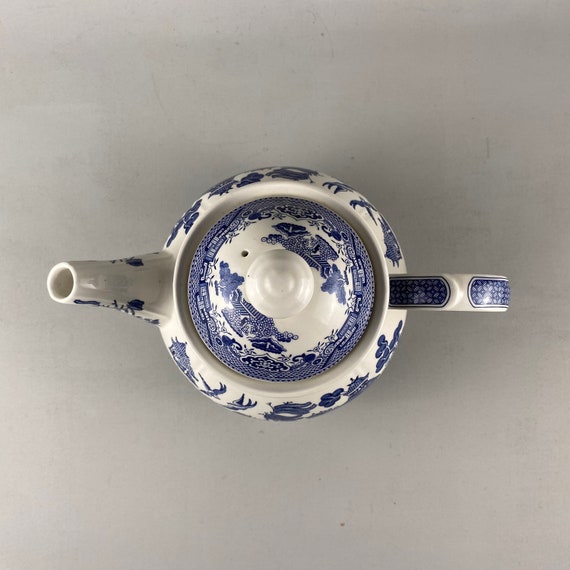This image captures a detailed, top-down view of a beautifully intricate teapot, reminiscent of traditional Chinese craftsmanship. The teapot, likely made from ceramic or porcelain, features a white base adorned with elaborate blue patterns that include flowers and architectural motifs. These decorations cover the entire surface, including the handle and the spout, which has a distinct open circle for pouring. The teapot's small, decorative lid also has a hole in it. The piece exudes artistic elegance suggestive of an ancient artifact or museum exhibit. The teapot sits on a subtly textured gray backdrop, possibly a tabletop or a cement surface, further emphasizing its ornate design.